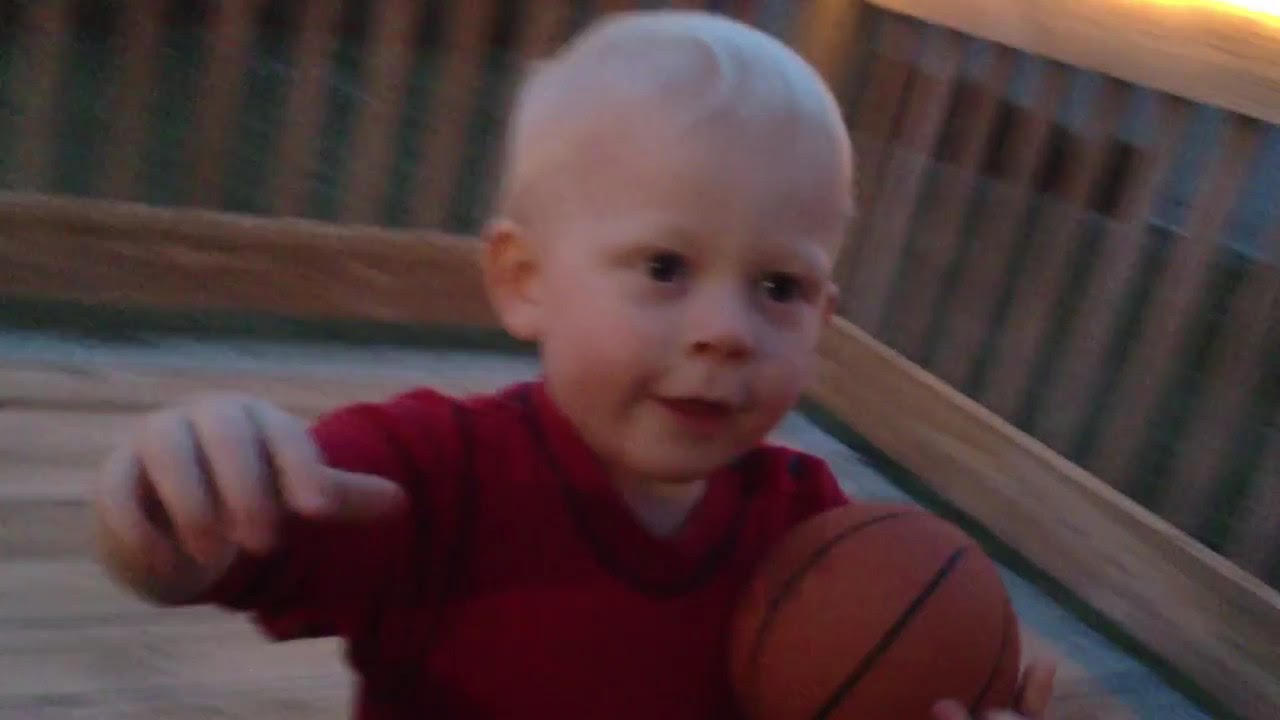This is a slightly out-of-focus, full-color photograph taken outdoors during the daytime. The roughly six inches wide by three inches tall image depicts a young Caucasian toddler, around one year old, with very fine, towheaded blonde hair and dark eyes. The boy is standing on a wooden deck or balcony, evidenced by the wooden railing with balusters. He is captured from the mid-chest up, wearing a short-sleeved red shirt. He holds a miniature orange basketball in his left hand, while his right hand is raised, fingers slightly drooped as if about to grab something. The toddler has a happy expression, with a partially open mouth hinting at a smile. In the background, between the railings, part of a blue structure, possibly a house or shed, and green grass from the yard are visible.